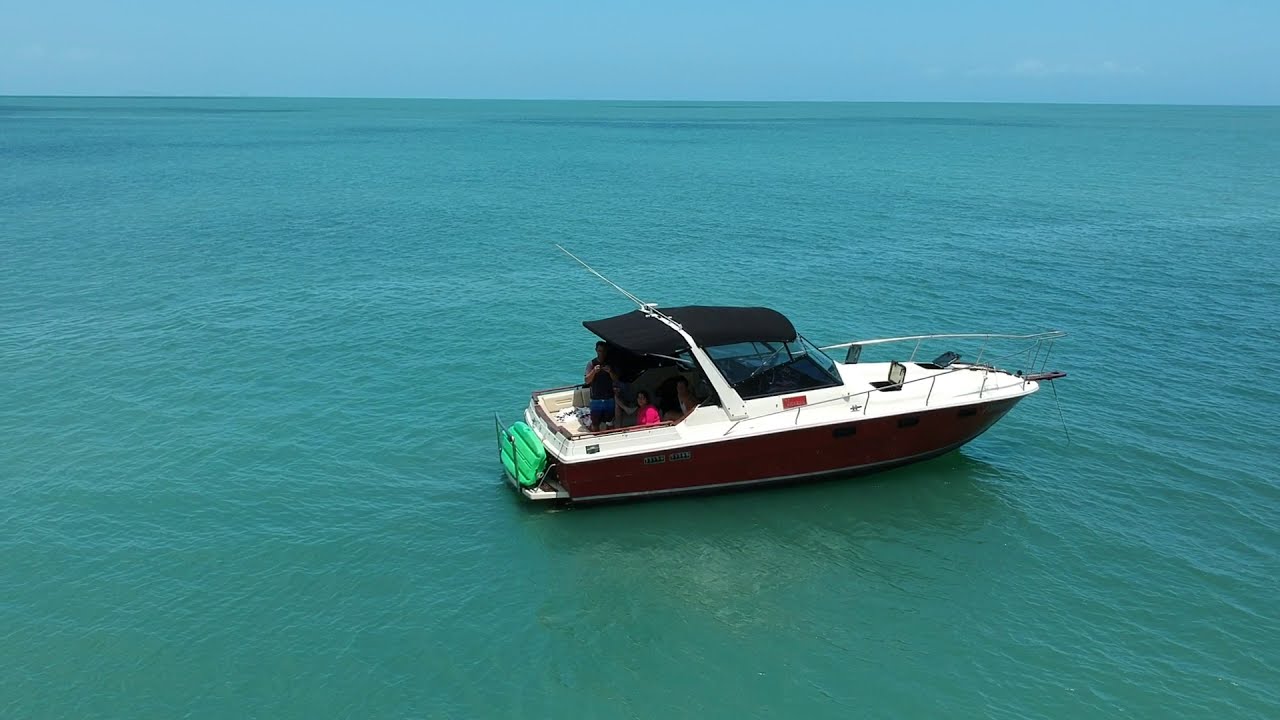From a slightly elevated vantage point, likely from a drone, the serene and expansive ocean stretches out in all directions under a clear blue sky, with no land in sight. The tranquil waters, a mesmerizing blend of blue and green, gently ripple beneath the sunlight. Anchored in the middle of this vast expanse is a small, personal fishing boat, approximately 25 feet in length. The boat's hull is burgundy on the bottom, transitioning to a white top, accented by a black fabric canopy. A single fishing pole is secured in a holder on the boat's railing. 

Onboard, a family of three enjoys their time at sea. A woman in a pink t-shirt gazes directly at the camera, which hovers just off the starboard side of the boat. Nearby, a man dressed in a black shirt and blue shorts is likely controlling the drone. The boat's deck features a green wakeboard stored neatly at the back. A small paddle boat is also docked at the rear. Visible textual details adorn the boat's side, adding an additional layer of character to the vessel. A rope extends from the bow of the boat into the water, securing it in place. The overall scene is both picturesque and serene, capturing a moment of peaceful leisure in the open ocean.